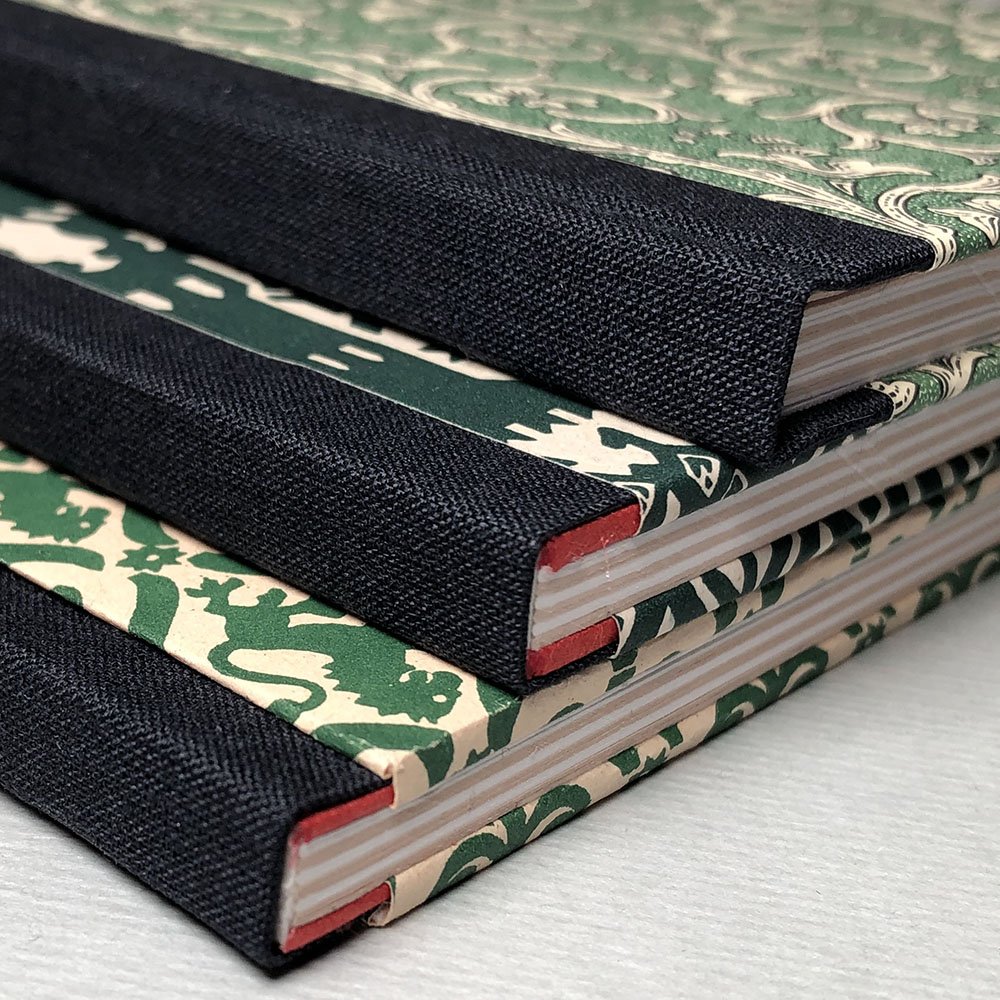This professionally photographed image showcases a close-up view of three ornate books, possibly diaries or ledgers, artistically stacked on a white surface. The books are not perfectly aligned but rather staggered, giving an intriguing stepped arrangement. Each book features a distinct, lavish cover design and a black fabric-like spine, adorned with red accents and textured patterns. The pages inside are alternating in tan and white. The top book is detailed in green with elegant golden curly Q designs. Beneath it, the second book is a darker green with lighter golden, bone-colored motifs. The bottom book stands out with its golden hue and green designs, featuring a motif that includes lion figures or symbols against a linen-like background. The exceptional lighting and focus in the photograph reveal the intricate details and textures of each book’s cover, capturing the essence of their craftsmanship.